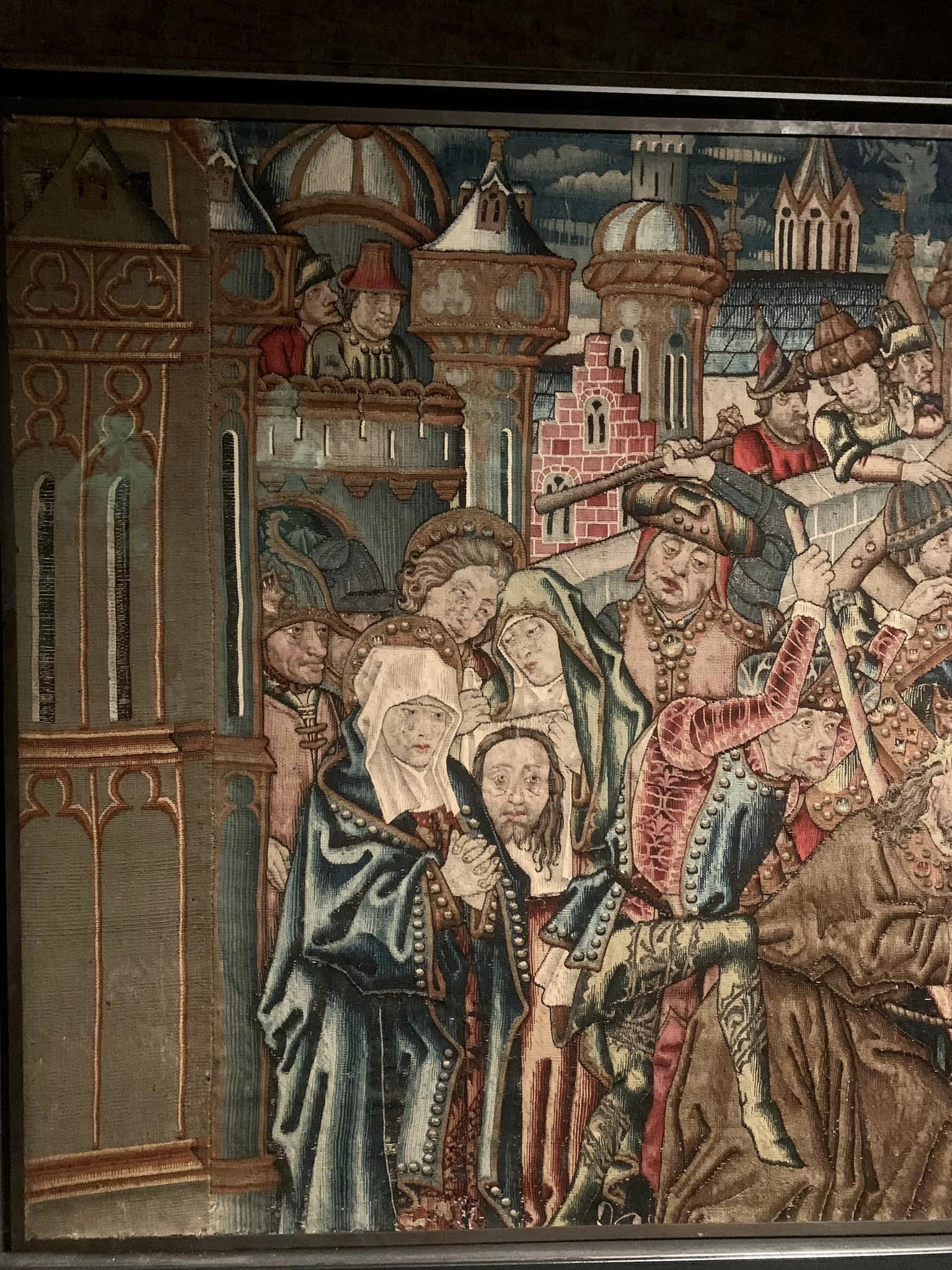This rectangular image, approximately five to six inches high and four inches wide, features an elaborate and colorful medieval or Renaissance-era painting. The upper portion of the image is framed by black borders on the top left and right corners, with a horizontal gradient of gray stretching across, transitioning from dark gray on the left to light gray on the right. Below this, a thicker stripe of gray metal acts as a base for the vivid scene below.

The painting depicts a bustling scene filled with richly dressed figures in classic European attire. The background reveals an array of castle structures with both pointed and domed peaks. On one ledge, men overlook a crowd gathered on the lower right side. This crowd includes solemn women, some with head coverings, one of whom holds a piece of paper or parchment displaying the image of a man with long brown hair, a mustache, and a beard.

Among the crowd, a dramatic scene unfolds: a man appears to be holding a pole, possibly signifying a violent act, while another man, perhaps an official, stands nearby in elaborate attire suggestive of royalty. A woman dressed in a blue cloak with a red dress underneath and a white habit, complete with a halo, stands to one side, possibly indicating sainthood. Another figure in the background also appears to be adorned with a halo.

The painting hints at a significant historical or religious event, with the beheading of John the Baptist being a potential subject. The overall atmosphere is dense with emotional weight, accentuated by the vibrant and varied colors of the characters' clothing.